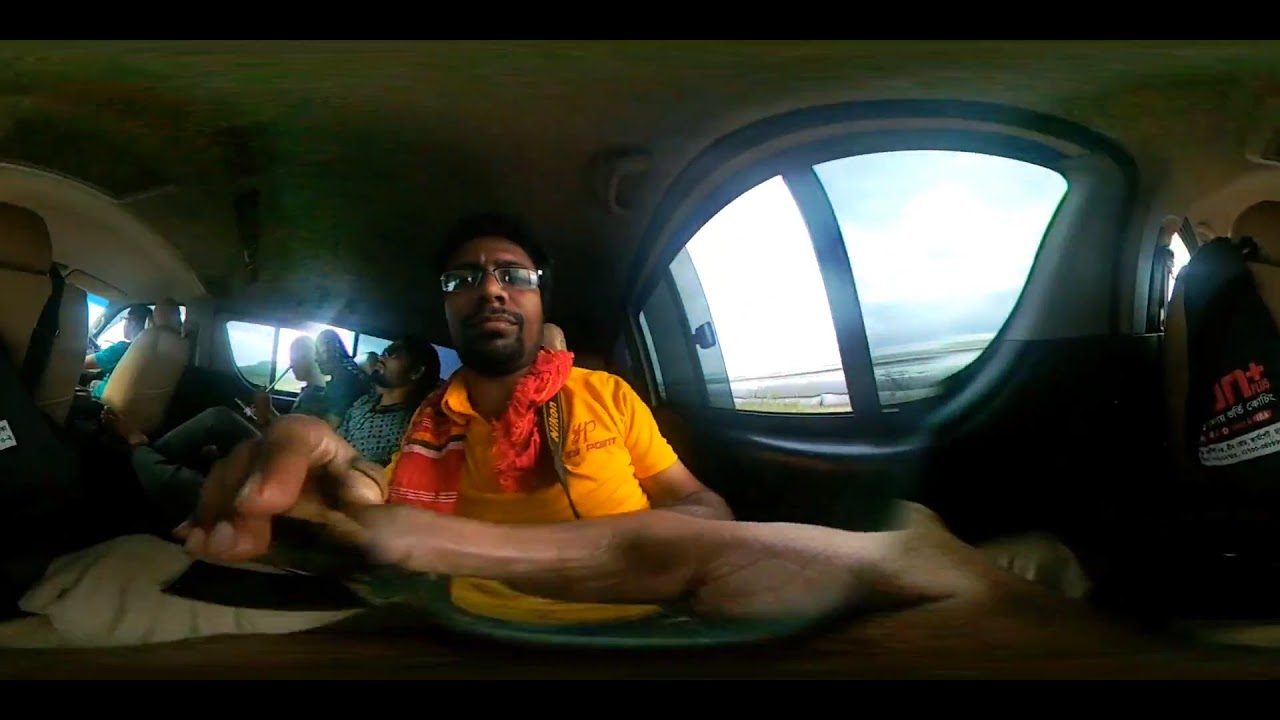In the image, a group of men are seated inside a vehicle, potentially an airplane, car, or bus, though it's difficult to determine the exact type of vehicle. In the foreground, a man is wearing glasses, a yellow collared shirt, and a red scarf. He has black hair, a goatee, and is looking directly at the camera, possibly recording himself. His hands are outstretched, possibly resting on another hand across the horizontal axis of the image. Beside him, another man in a short-sleeved green shirt and glasses is seated in the front passenger seat. In the back seat, three other men are seated; one man's head rests against the seat, while the other two look forward. The windows next to these men are open, revealing a gray sky outside. The vehicle's front seats are leather, either cream, brown, or beige. The foreground of the image appears slightly blurry, adding a sense of depth to the scene.